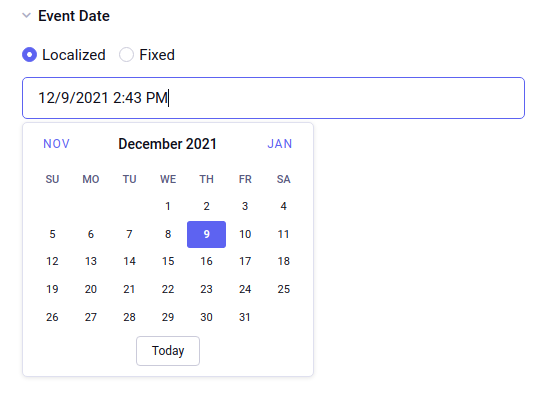The image features a user interface with a white background. At the top, there is a dropdown button labeled "Event Tab." Below this dropdown, there are three radio buttons: one labeled "Localize," another labeled "Fixed," and the third labeled "Localize Event Selected," with the last option highlighted in blue. Underneath these radio buttons, there is a blue-bordered text box displaying the date and time as "12/9/2021, 2:43 PM."

Below this section, a calendar for December 2021 is displayed, flanked by navigation options for "November" on the left and "January" on the right. The calendar layout includes seven columns for the days of the week: Sunday, Monday, Tuesday, Wednesday, Thursday, Friday, and Saturday. The first day of December is shown to be a Wednesday, and the last day, the 31st, falls on a Friday. No dates from the preceding or following months are included.

The calendar is outlined with a light gray border, and at the bottom, there is a white button with a gray border and the text "Today" in black, centered within the button. The rest of the interface is set against a plain white background.